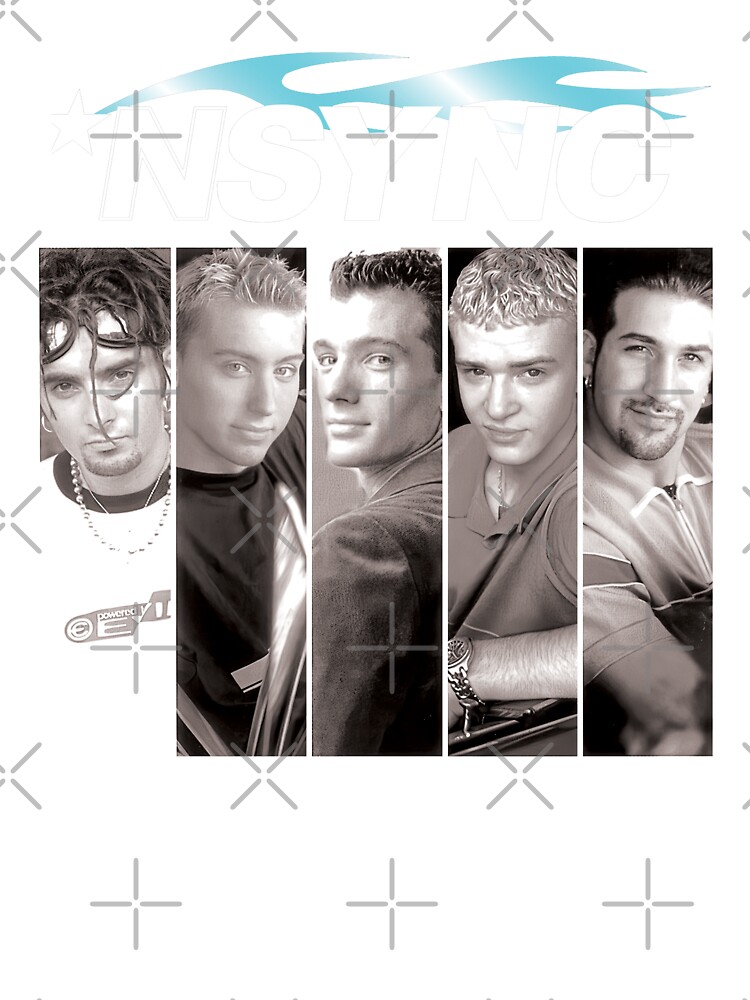This detailed image features a photo collage showcasing the five members of the iconic NSYNC boy band. Set against a predominantly white background adorned with plus signs and X's in light gray, the word "NSYNC" is subtly outlined in light gray at the top, creating an almost invisible yet distinctive label. Each of the five band members is presented in vertically long, narrow black-and-white photographs that exude a vintage feel with a subtle brownish tone. The band members are aligned from left to right, starting with a dark-haired man on the left who has longer hair, an earring, and a goatee. Notably, the far left and far right members sport goatees, with the far-right man having a unique dreadlock hairstyle. Most members have dark hair and are dressed in darker tops, staring straight ahead with faint smiles, except for the far-right individual who stands out with a more reserved expression. Above the photos, a blue strip or wave-like design accents the collage, contributing to the overall theme. This stylistic representation serves as an evocative advertisement for the NSYNC band, capturing their youthful, energetic aura in a single, cohesive visual.